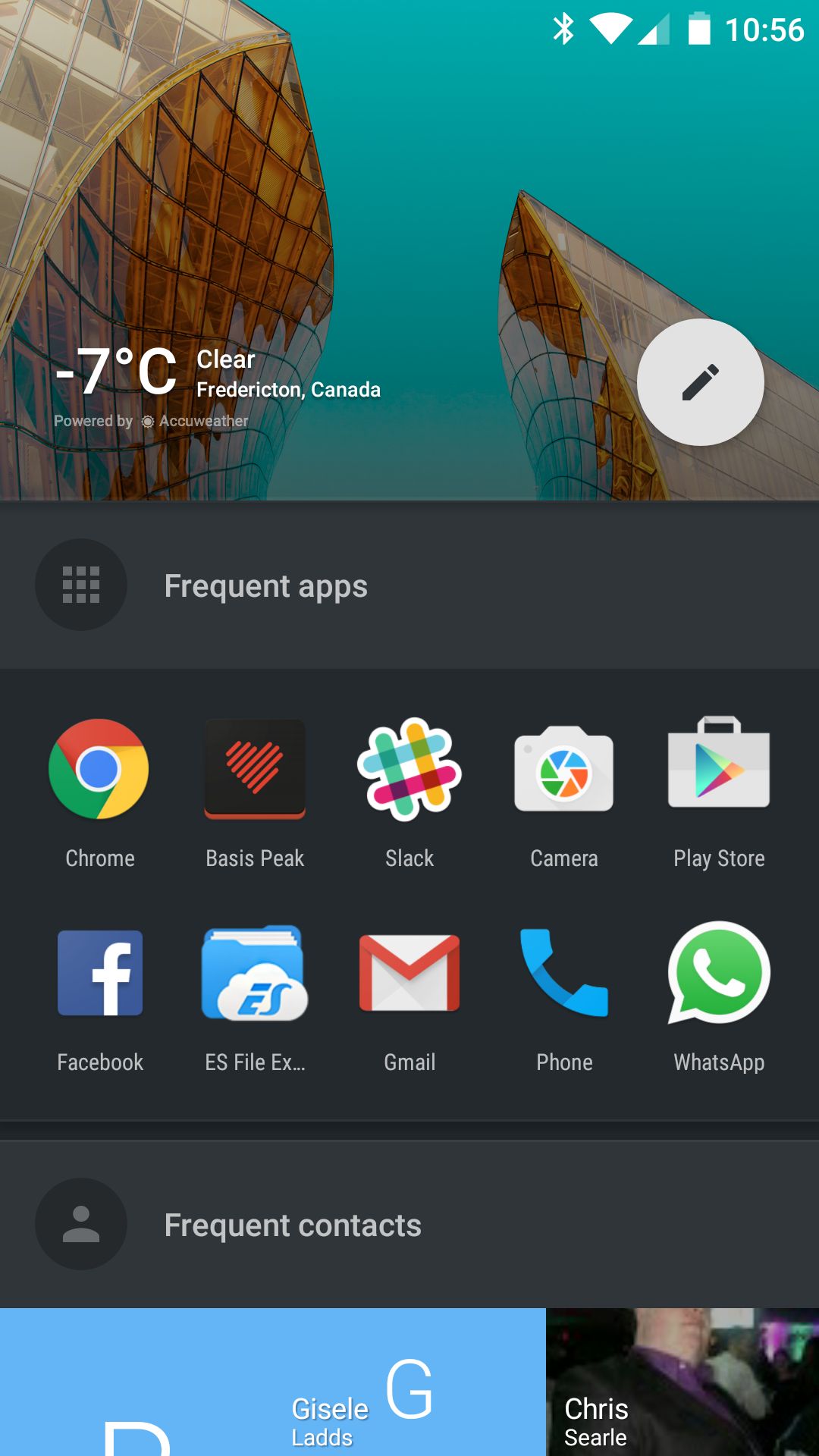This image is a screenshot of a smartphone home screen, showcasing a detailed and visually striking wallpaper. The background image is of a modern, glass-clad building featuring curving, wave-like facets, reminiscent of a design by the Guggenheim, with glass tinted in an amber hue. The sky in the background has an unusual greenish tint. 

On the upper left side of the screen, there is weather information displayed in white text, showing "-7°C, clear in Fredericton, Canada," powered by AccuWeather. To the right of the weather information is an icon of a pen inside a white circle, which suggests an option to edit or customize the home screen.

Below the wallpaper, a gray overlay pop-up titled "Frequent Apps" shows a grid of ten applications arranged five across and two down. The first row includes icons for Chrome, BasisPeak, Slack, Camera, and Play Store. In the second row, there are apps for Facebook, ES File Explorer, Gmail, Phone, and WhatsApp.

Additionally, there is a lighter gray panel labeled "Frequent Contacts." This section prominently displays a contact named Giselle Lads on a blue background, taking up about two-thirds of the section. To the right, a smaller section features a photo of a man labeled Chris Cyril. The arrangement suggests they might be part of a horizontal scrollable list.

The overall layout and details, including the unique wallpaper and specific app and contact selection, provide a personalized and distinctive view of the user's smartphone interface.